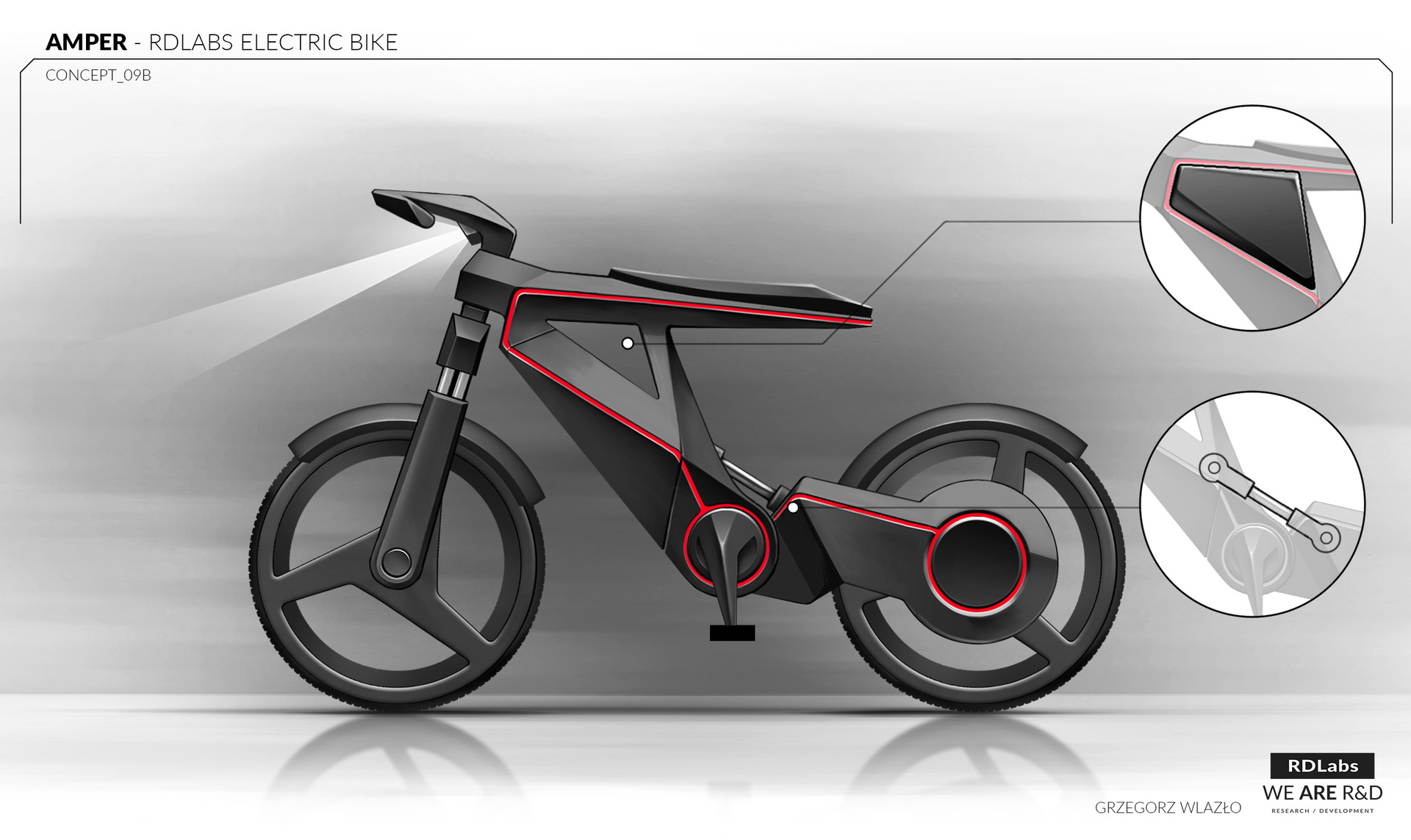This is a detailed digital concept illustration labeled "Amper RD Labs Electric Bike" at the top left corner with the text "Concept 09B" beneath it. The bike features an innovative, futuristic design with a sleek black frame accentuated by red highlights. It sports an elongated, platform-like seat and ergonomic wheels that lack traditional spokes, instead featuring three structural bars connecting to the wheel's rim. The handlebars are streamlined with an integrated headlight pointing forward but slightly downward. Various components of the bike are highlighted with gray and red lines, including a reflective portion and the area around the pedals, highlighted by two zoom-in circles on the right. The background is a gradient of gray and white, and the bike appears to be mounted on a platform reflecting its sophisticated style. At the bottom right, the text "Audi Labs. We are R&D, research developments," along with the name "Grzegorz Wlazlo," is inscribed, adding a professional touch to this cutting-edge design blueprint.